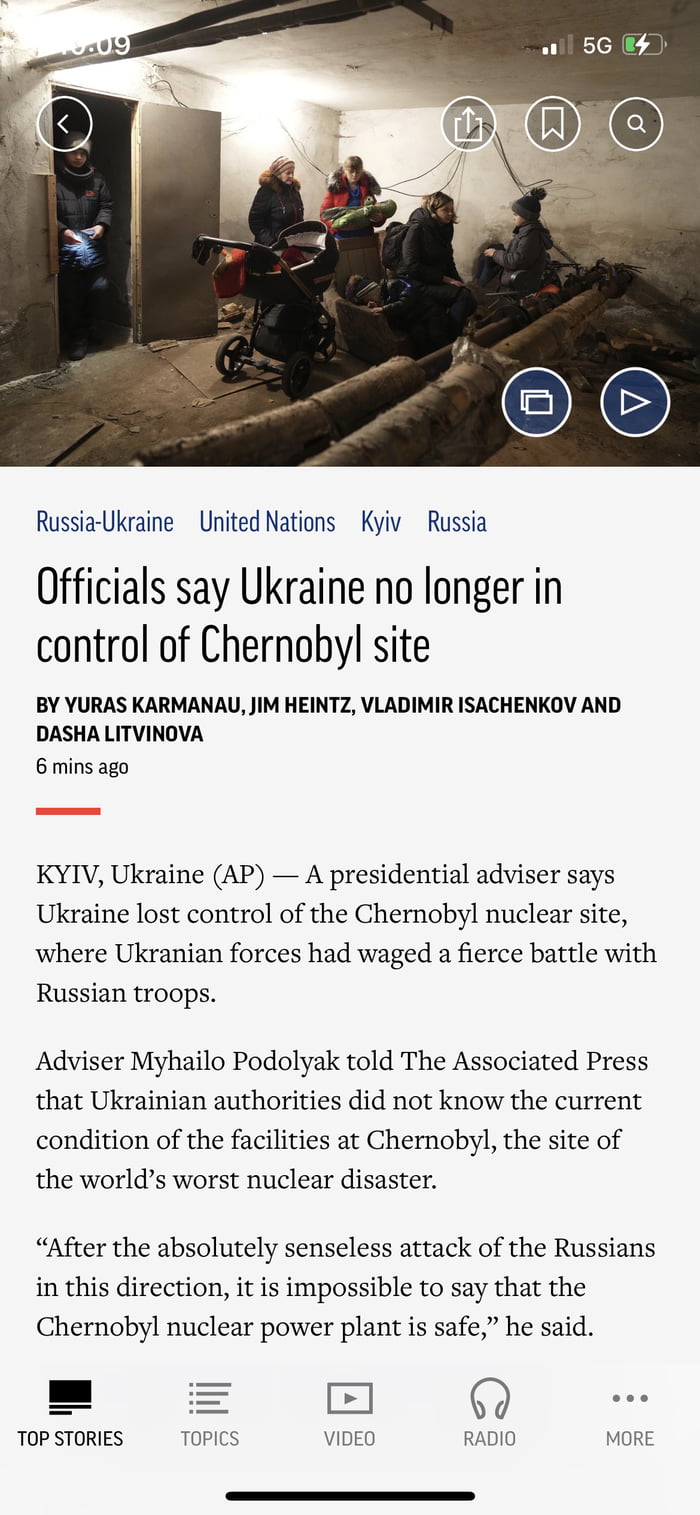The image displays a news website interface. At the very top, there is a realistic photograph that depicts a darkened room with concrete walls and several pipes. In the scene, multiple people are shown, along with a carriage and a door through which someone is seen walking. Overlaying the photo is text that reads "10:09" in white print, along with icons indicating battery life, 5G connection, and cell signal strength.

Below the image, the headline reads: "Russia, Ukraine, United Nations - Kyiv, Russia. Officials say Ukraine no longer in control of Chernobyl site." The text is presented on a gray background and includes the authors' names and the posting time. Further details reveal that, according to a presidential advisor, Ukraine has lost control of the Chernobyl nuclear site, where intense fighting with Russian troops took place. The advisor, Mihailo Podolyak, informed the Associated Press that Ukrainian authorities are currently unaware of the status of the Chernobyl facilities, which is significant as it was the site of the world's most catastrophic nuclear disaster. Podolyak commented that due to Russia's "absolutely senseless attack" in that direction, it is no longer possible to guarantee the Chernobyl nuclear power plant's safety.